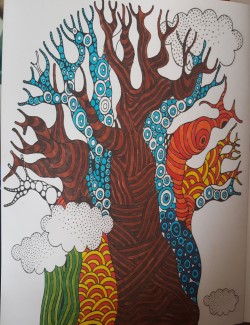This image depicts a hand-drawn artwork on a small piece of white paper, featuring an artistic representation of a baobab tree reminiscent of the iconic tree from "The Lion King". The drawing is created using black pen for outlining and various colored markers to fill in details. The tree's trunks, which are intertwined and attached to each other, showcase intricate crisscross and swirling patterns. These trunks are vividly decorated with sections of brown, yellow, red, blue, and white. Extending upwards, the trunks culminate in stylized leaves that resemble white clouds adorned with dots, giving the tree a whimsical and imaginative appearance. The overall effect is a vibrant and intricate piece that captures the essence of a baobab tree through a kaleidoscope of colors and patterns.